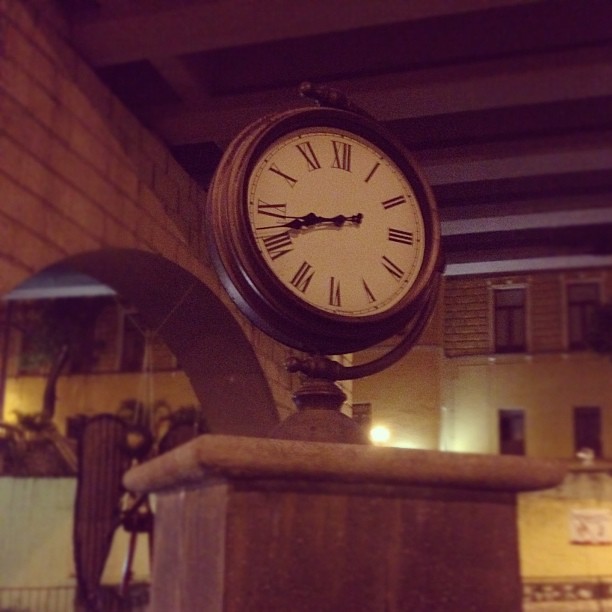This image captures a meticulously crafted vintage clock with a robust steel construction, prominently displayed atop a concrete pedestal in a restaurant interior. The clock features a white dial face adorned with Roman numerals, providing a touch of classic elegance. The outer case of the clock is notably thick, complemented by a semicircular steel arch that partially encircles the right half of the clock, adding to its unique design. The backdrop reveals an arched entryway, enhancing the architectural aesthetic of the setting, along with several paintings depicting buildings, which lend an additional layer of artistic flair to the scene.